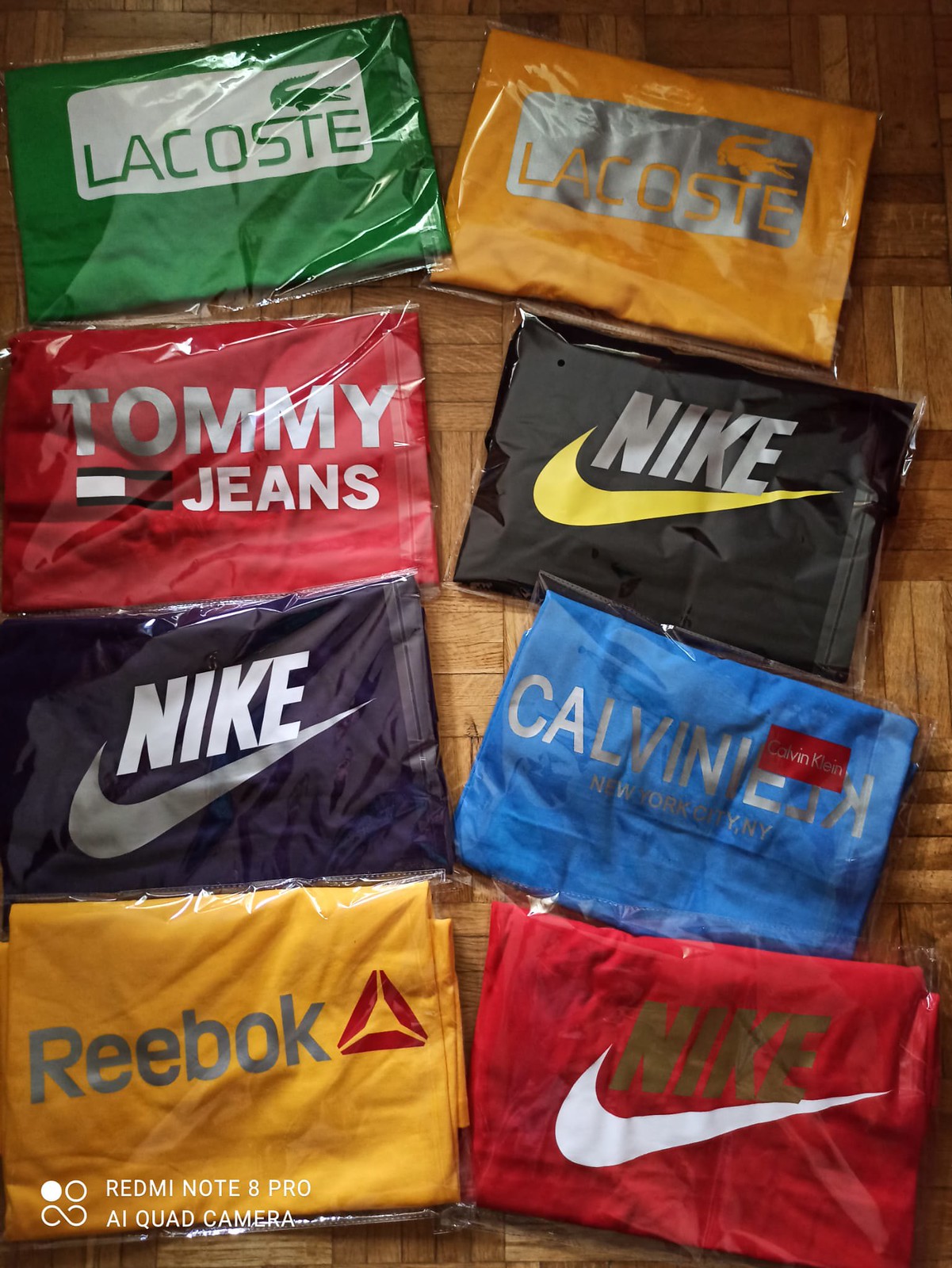This photograph depicts eight clear plastic bags, each containing a folded t-shirt, arranged in two rows of four on a brown hardwood floor with a distinct squared tile pattern. The t-shirts showcase vibrant colors and the logos of well-known brands. From left to right, the top row displays a green Lacoste t-shirt featuring the signature green alligator emblem, an orange Lacoste shirt with a silver rectangle and logo, a red Tommy Jeans t-shirt with bold white lettering, and a black Nike t-shirt with a yellow swoosh. The bottom row includes a purple Nike t-shirt with a silver swoosh, a blue Calvin Klein t-shirt with backward "CALVIN KLEIN" text and "New York City, New York" written below, a yellow Reebok t-shirt with a gray logo and red symbol, and a red Nike t-shirt with brown "Nike" text and a white swoosh. A watermark in the bottom left corner reads "Redmi Note 8 Pro AI Quad Camera," accompanied by a white logo resembling two circles above a sideways S.